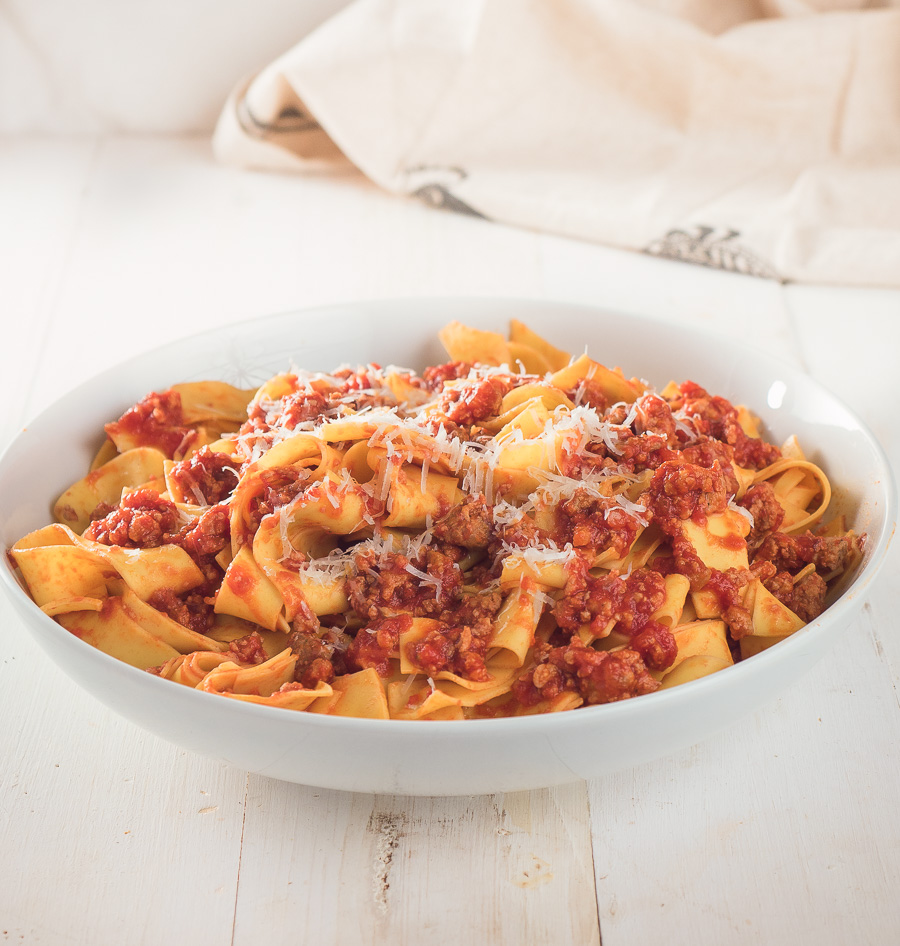The image displays a white, shiny bowl filled with pasta, likely ziti, placed upon a light wooden surface. The pasta is covered in a rich red tomato sauce that contains chunks of ground meat. The sauce, which appears to be somewhat fried, is generously topped with shredded cheese, possibly cheddar. The noodles look fresh and slightly eggy. The background includes a white cloth, adding a touch of elegance to the scene. The overall color palette of the image is dominated by shades of white, cream, yellow, and vibrant red.